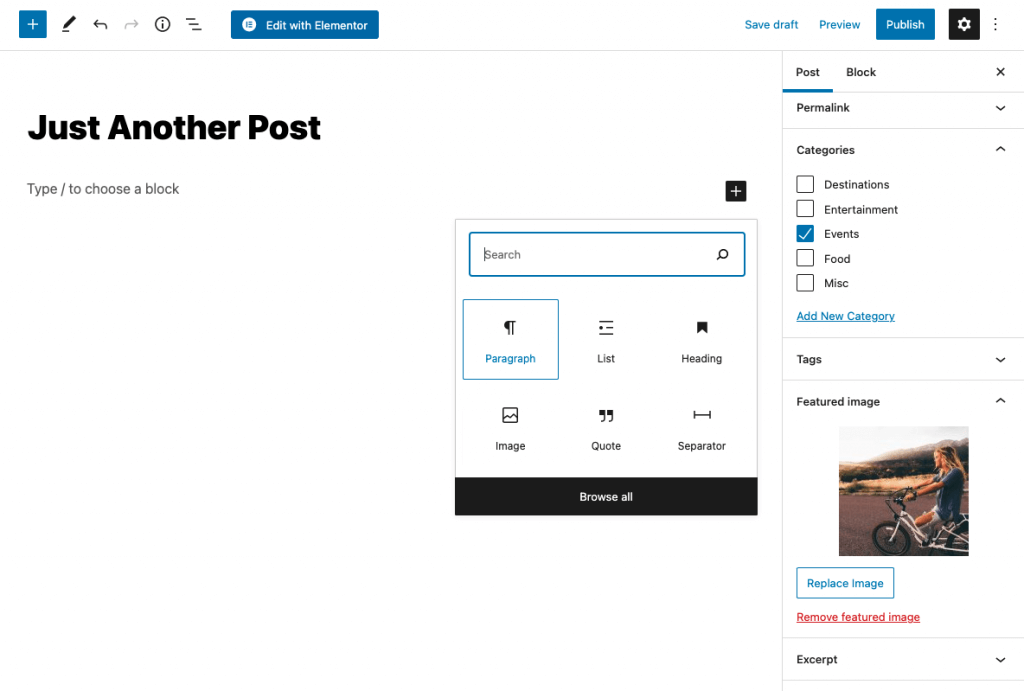The image depicts a user interface of a web-based professional publishing and editing platform, likely focused on blogging or article writing. At the top of the page, there is a navigation area with options such as "Edit with Elementor" and a back button. The top right corner features a "Publish" button, indicating the functionality to finalize and share the content. The main workspace displays a prompt stating, "Type forward slash to choose a block," offering various page elements like paragraph, list, heading, image, quote, and separator. On the right side, there's a pane with two tabs: "Post" and "Block," with the user currently in the "Post" tab. They are seen interacting with the categories section, having selected "Events" as the category for their post. Additionally, the post contains a stock photo of a person riding a motorcycle, illustrating the platform's capability to add pre-uploaded images without needing external sources. Overall, the platform provides a comprehensive environment for creating, categorizing, and publishing blog posts or articles easily.